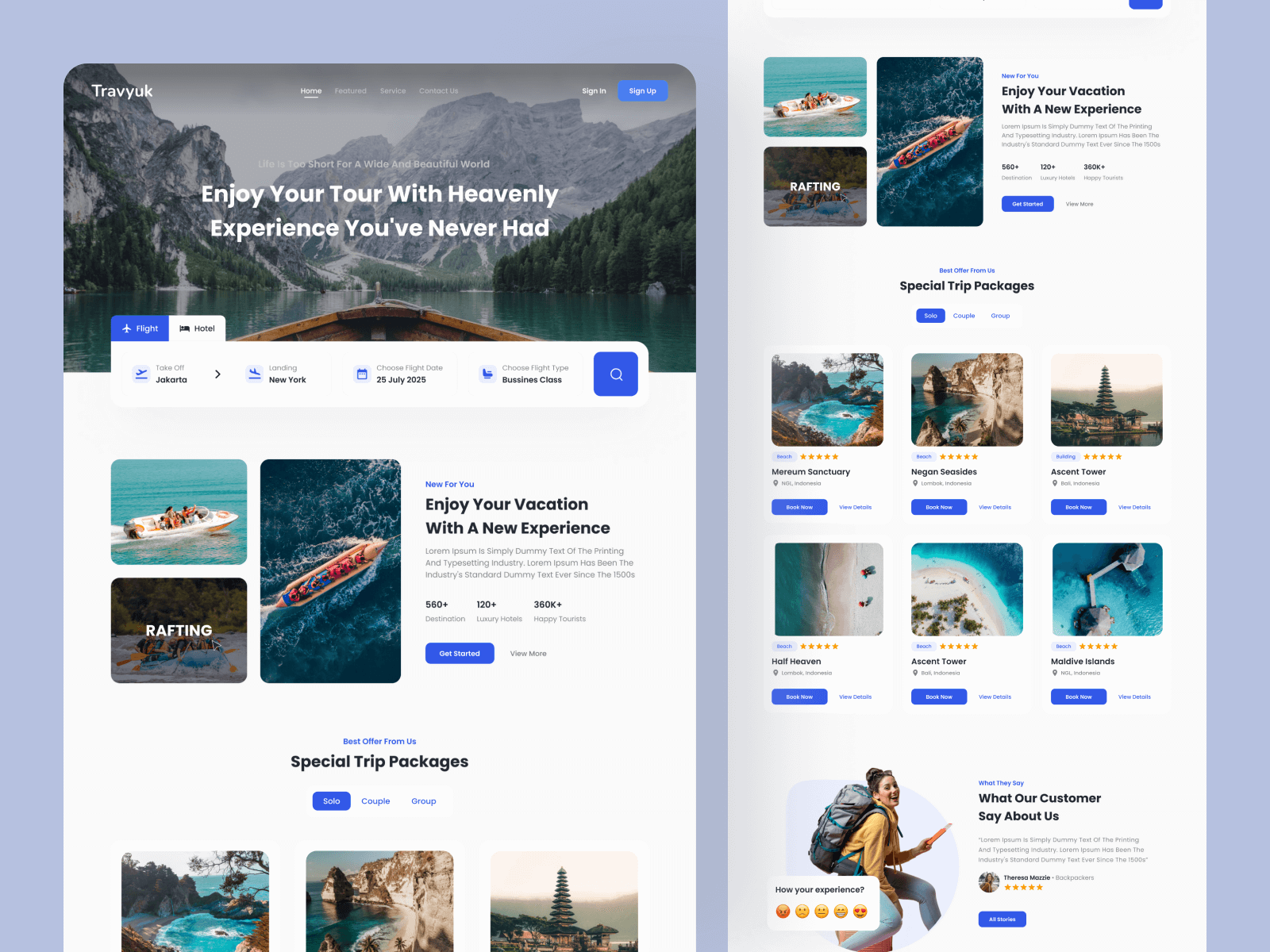**Caption:**

The image showcases an advertisement for Travelin, prominently displaying "Trav-Yuk" in the top left-hand corner on what appears to be their homepage. At the center of the header is a highlighted title on the menu bar, featuring four selections whose names are obscured. A blue "Sign In" or "Sign Up" button is situated on the right-hand side.

Dominating the central area of the page is a bold statement: "Enjoy your tour with Travelin - an experience you have never had." This text is set against a white background. Below this, two labels are present, one depicting a plane and the other, partially obscured.

Further down the page, there are several media images, including boats. An additional message reads: "Enjoy your vacation with a new experience" in black text, accompanied by a brief paragraph. Beneath this section, the text “Special Trip Packages” heralds two rows of images. The first row displays three pictures, and to the right of this, another set of three similar photographs, visually echoing the initial set. All imagery extends down to the bottom of the page, emphasizing the advertised travel experiences.